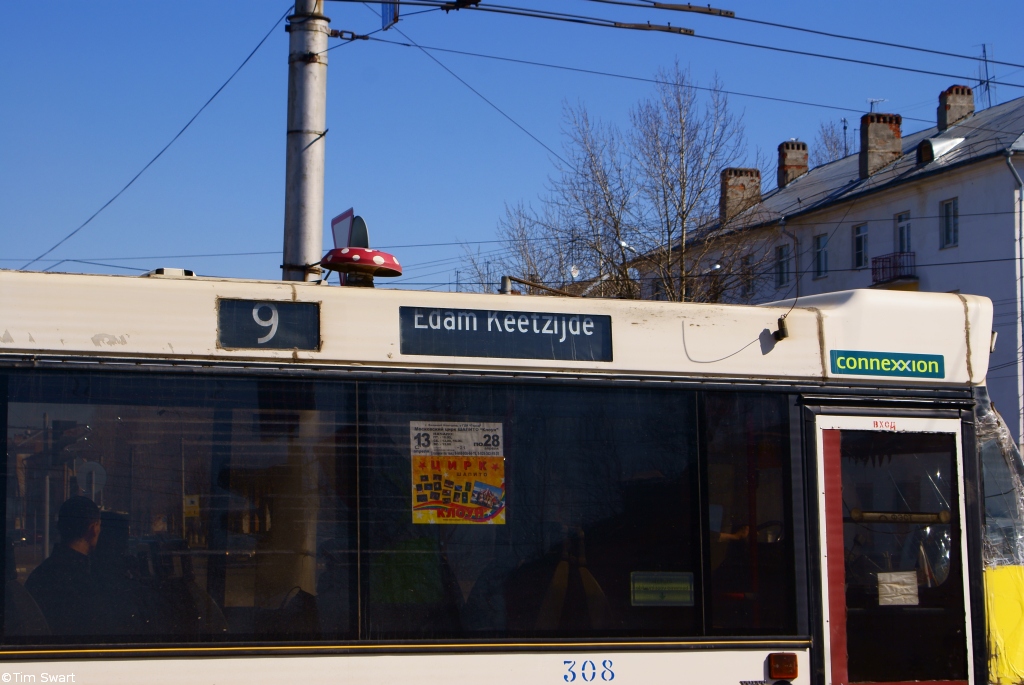In this vibrant daytime photograph, a large white transit bus with tinted windows dominates the foreground, stretching from the left to the right edge of the image. A striking red strip accents the door, and an advertisement displaying the word "Jumper" is visible on one of the windows. Notably, the bus is marked with the numbers 308 and 9, possibly indicating the route and bus number. 

The serene, cloudless sky is a brilliant blue, providing a vivid backdrop. Barren trees, devoid of leaves, frame the scene with their intricate network of branches and twigs. Behind the bus, tall European-style architecture, possibly from the Netherlands, rises into view, featuring numerous windows and balconies, suggesting a residential complex or apartment building. A silver telephone pole with power lines extends above the bus, adding to the crisp, detailed composition of this wintertime scene.